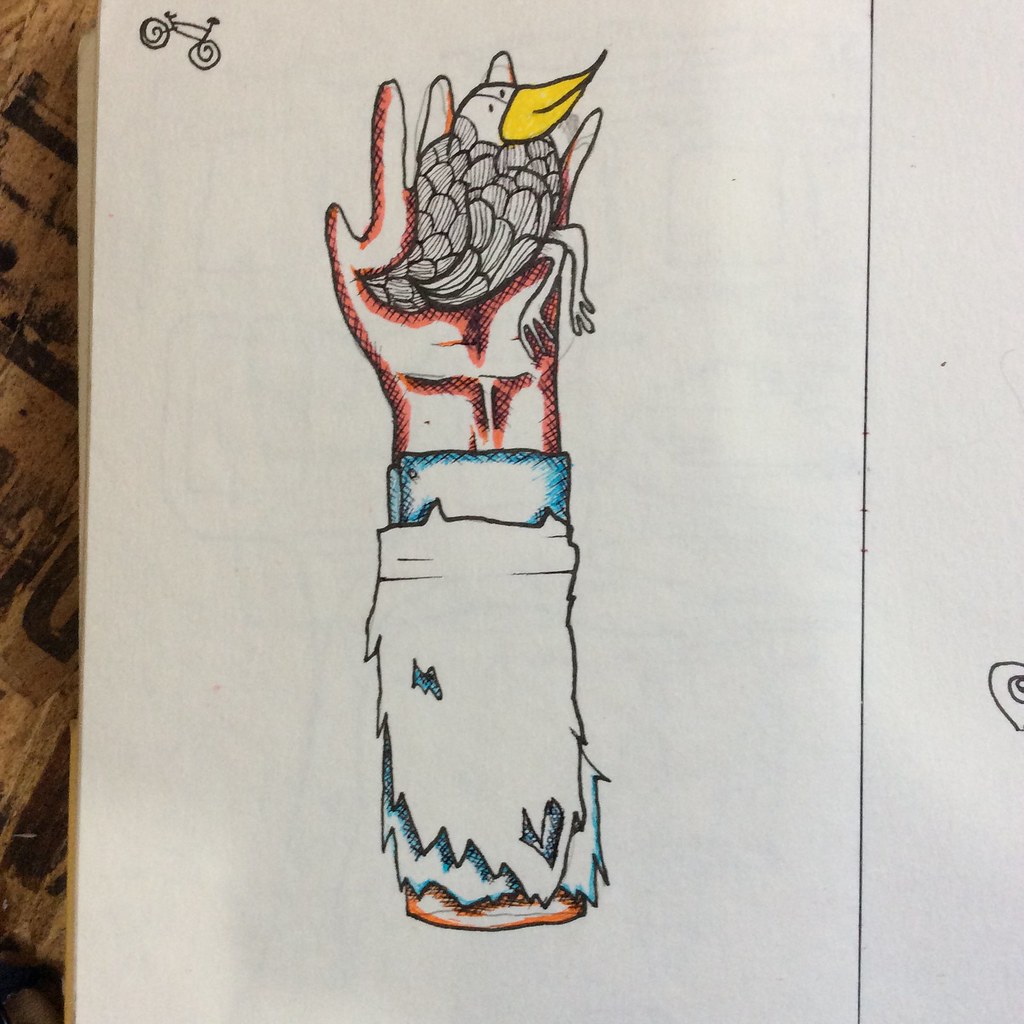The image features a colored ink drawing on a vertically oriented, white piece of paper that appears to be part of a notebook, identifiable by a spiral ring peeking out on the right edge. The left side of the paper features a small black ink sketch of a bicycle. The central illustration depicts a disembodied arm severed above the elbow, with the stump displaying a clean cut free of blood or veins. The arm is covered in tattered, white fabric with visible holes and a jagged blue-outlined sleeve. The hand, outlined in red and black, cradles a bird. The bird has a white head, a yellow beak, black and white feathers, and two white legs. The bird's legs extend over the pinky side of the hand, revealing three small toes. The background shows mingled light and dark brown hues, giving the drawing depth and contrast.